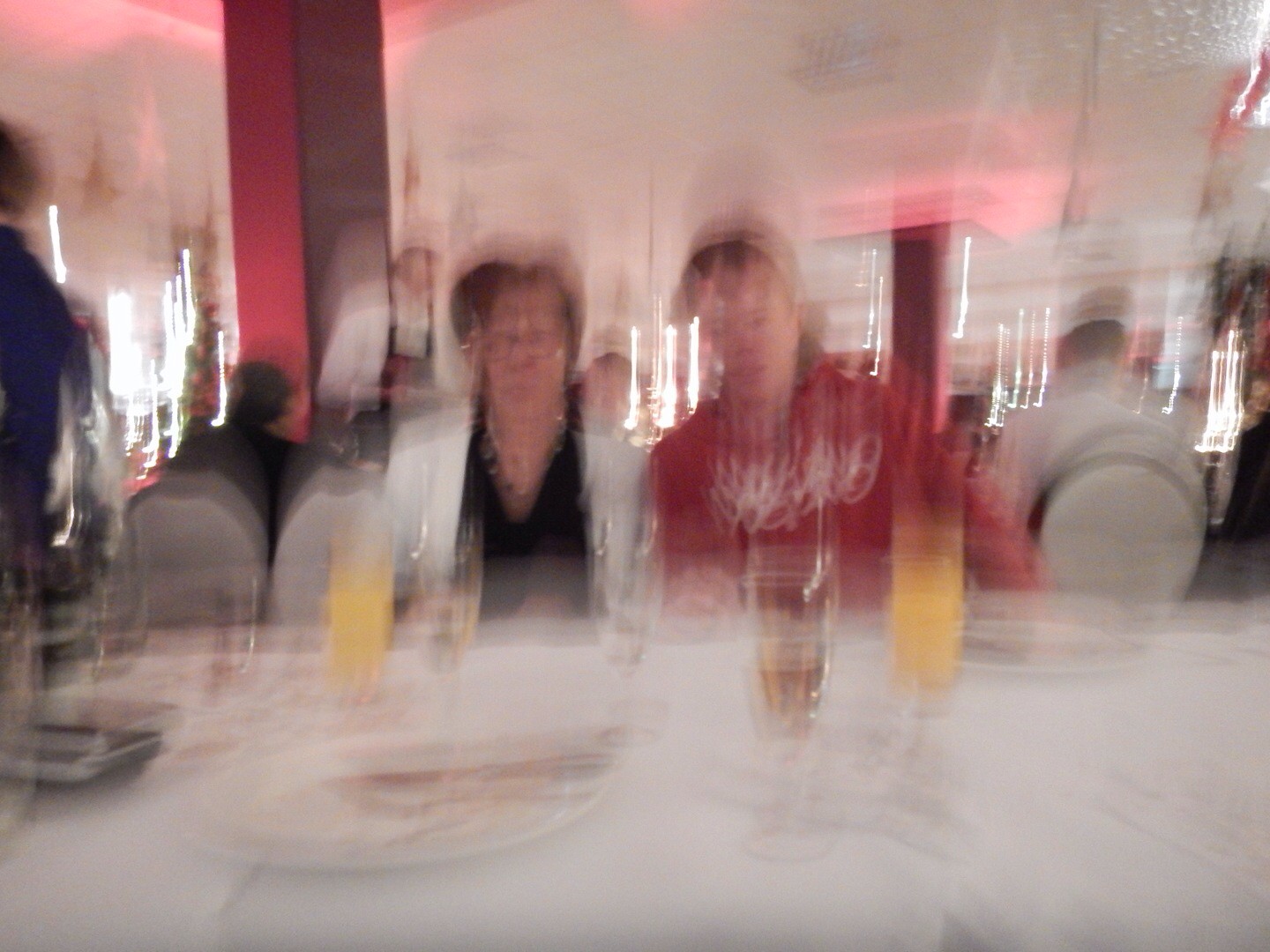The photograph is a heavily blurred indoor scene in a landscape orientation, depicting what appears to be a mother and son dining at a high-end restaurant. The entire image suffers from significant motion blur, which causes an elongated, vertical ghosting effect across all elements. 

The dining setup features pristine white tablecloths adorned with elegant bone china plates and silver cutlery. There's a variety of glassware on the table, including wine glasses with a brownish liquid and juice glasses filled with orange juice, which appear to have streaked upward due to the camera movement. A candle and a phone are also visible among the table items. 

The woman, seated on the left, is dressed smartly in a black V-neck top under a white, open suit jacket, accessorized with a necklace and glasses. The young man next to her, on the right, is wearing a red hooded top with graffiti-style white writing on the chest. The background reveals a server in a long-sleeved white shirt and dark apron, and other patrons seated at tables, with one noticeable figure in blue walking to the left. The room is characterized by a white ceiling supported by large red pillars. Despite the lack of sharpness, the setting suggests a sophisticated and possibly cruise-ship dining experience.